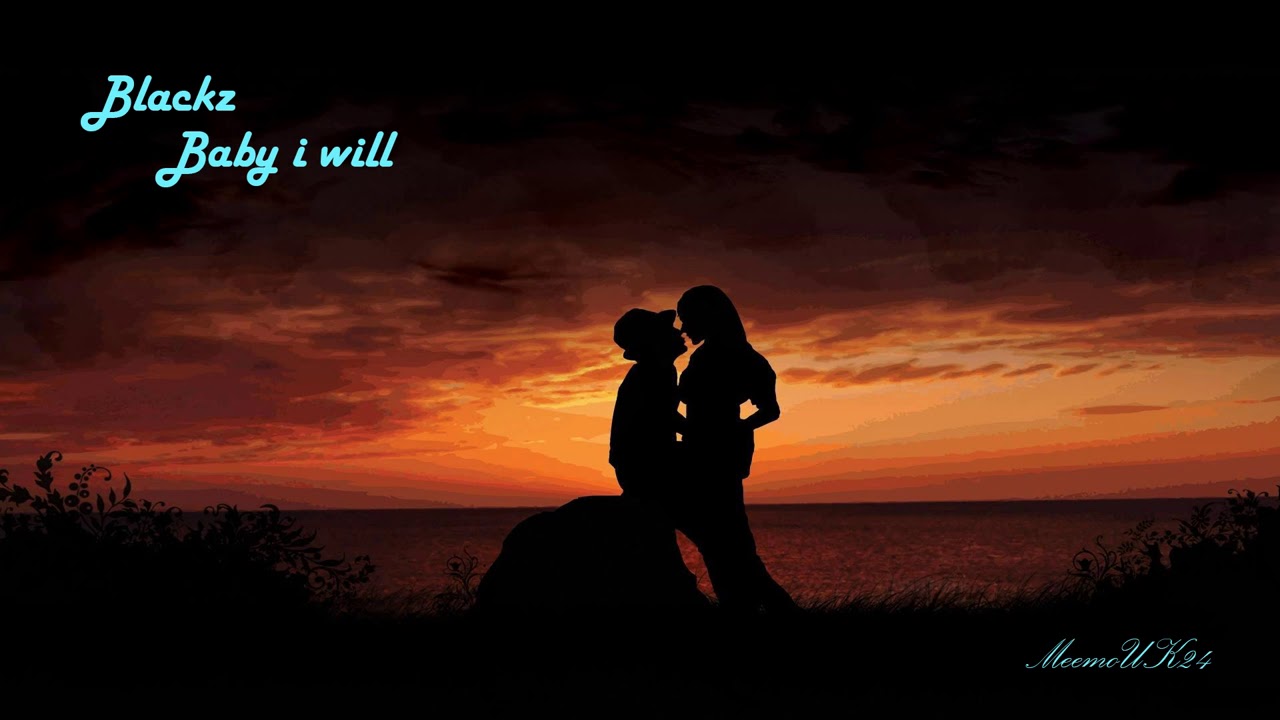This atmospheric graphic image, possibly a digital artwork, portrays the silhouette of a man and a woman, seemingly on the verge of a kiss, their noses almost touching. Set against a dramatic sunrise or sunset, the colors transition from deep blacks at the top and bottom of the image to vibrant oranges and yellows near the horizon, reflecting subtly on a tranquil lake in the backdrop. The centered figures, leaning against a rock with the man donning a hat, evoke a moment of intimate connection. In the upper left corner, blue script text reads: "Blacks, baby I will," with the distinctive spelling B-L-A-C-K-Z. The lower right corner features a signature also in blue, which appears to say "MIMO UK 24." The entire scene is framed within a horizontally oriented rectangle, enhancing its picturesque quality.